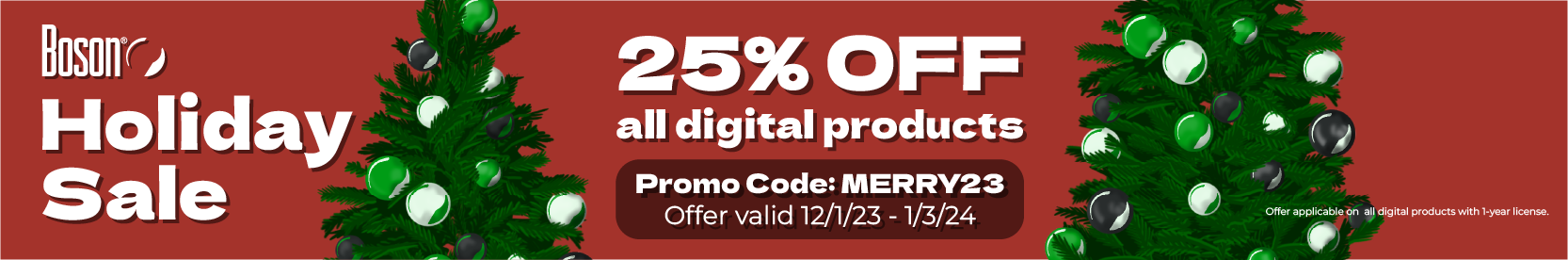Here is a refined and detailed caption for the image:

"A festive red banner featuring a Christmas theme announces a holiday sale. On the left side, in white text, it reads 'Bosson,' with 'Holiday Sale' in larger white letters directly below. A partially visible green Christmas tree adorned with ornaments extends from the top to just above the middle, flanking the left and right sides of the banner. At the center of the red banner, bold white letters proclaim '25% off,' with 'All Digital Products' written in smaller white text beneath. A maroon-colored section at the bottom contains the text: 'Promo Code: MERRY23' in capital letters. Below that, it states, 'Offer Valid: 12/1/23 - 1/3/24' in a thinner white font. The right side of the banner mirrors the left with the middle part of the decorated Christmas tree, though there is some small, indecipherable writing along its edge. The entire banner measures approximately an inch in height."